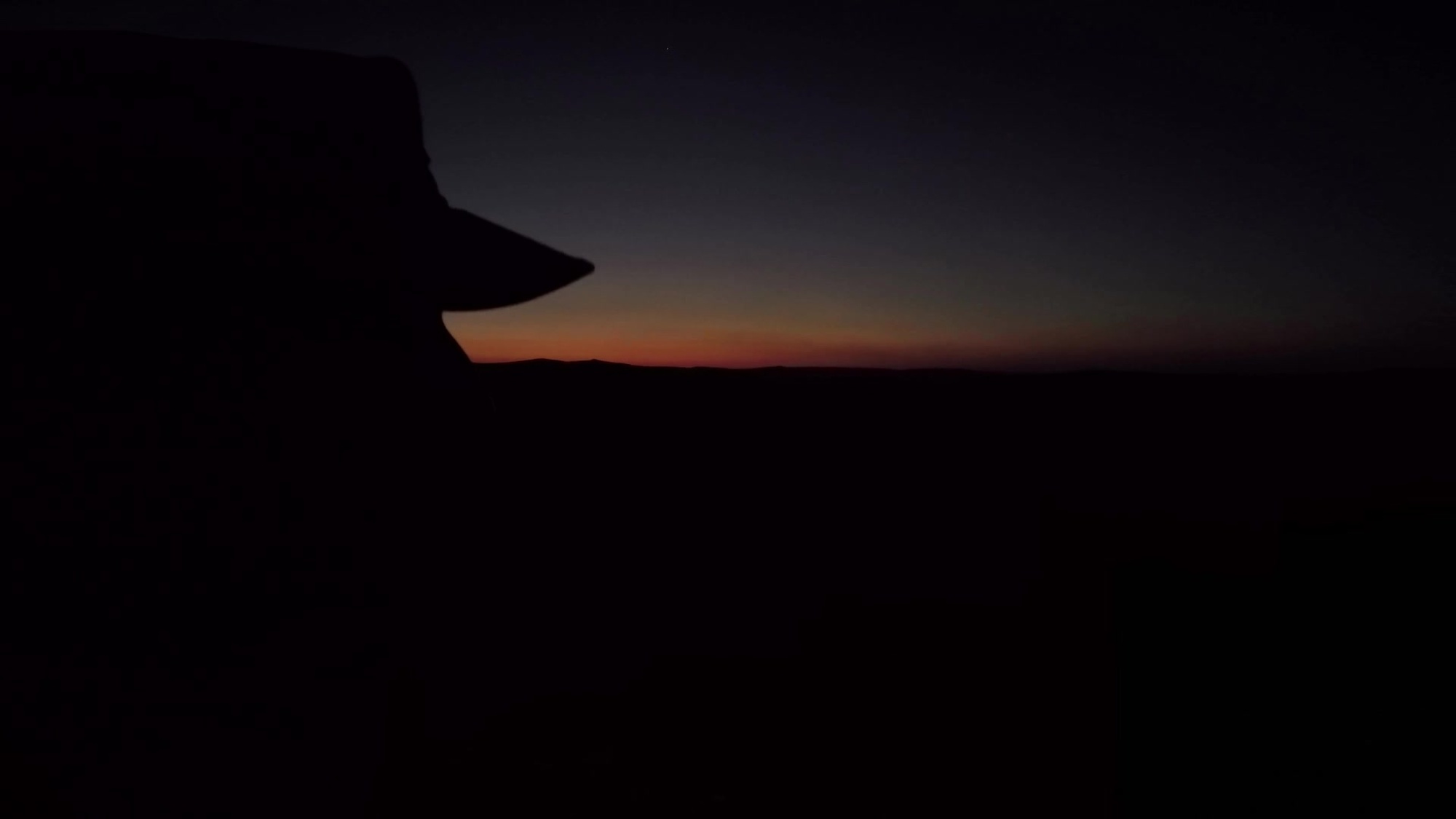This photograph depicts an outdoor scene captured in the very dark twilight, where the sun has almost completely set. The majority of the horizon and foreground are shrouded in deep black, possibly indicating the presence of mountains or natural structures that obscure any further details. Above the horizon, a gradient of fading light reveals layers of colors: a deep blue at the top transitioning into a faint blue, followed by a greenish tint, then a yellow layer, and finally a gradient from red to a muted purple near the horizon. On the top left side, a silhouette resembling the side of a hat is visible, hinting that the photo might have been taken from behind someone wearing a hat. The overall scene hints at the tranquil end of the day, with only the colorful sky and indistinct silhouettes breaking the darkness.